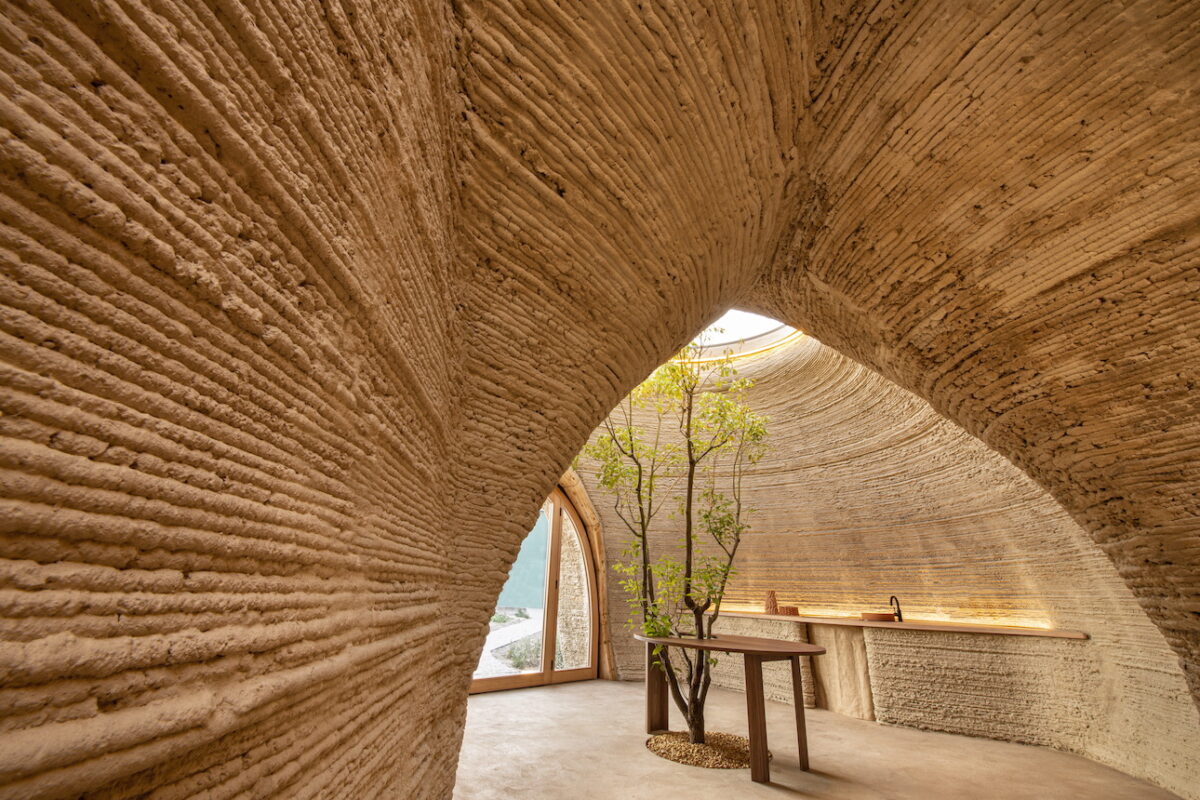The image depicts the interior of a unique, modern cave-style house with a striking, new-age architectural design. The walls and ceiling are crafted from intricately patterned clay or rock, giving them a textured, corrugated appearance. The structure's shape is a mix of a triangular and dome-like form, with an upside-down V-shaped doorway leading to another section of the room. A central skylight at the apex of the dome allows natural light to flood in, illuminating a tree that grows through a bean-shaped wooden table positioned beneath the skylight.

To the right side of the room, there's a wall-mounted wooden shelf and an illuminated area that may be a sink with a faucet and a brown bowl. The floor is made from smooth, textured wood, providing a contrasting surface to the earthen walls. An oval-shaped window with a rounded top and straight bottom offers a view of what appears to be a road or sidewalk, and another partial window is visible along the wall, perhaps showcasing a glimpse of water. The space blends organic elements with innovative design, creating a harmonious and inventive living area.